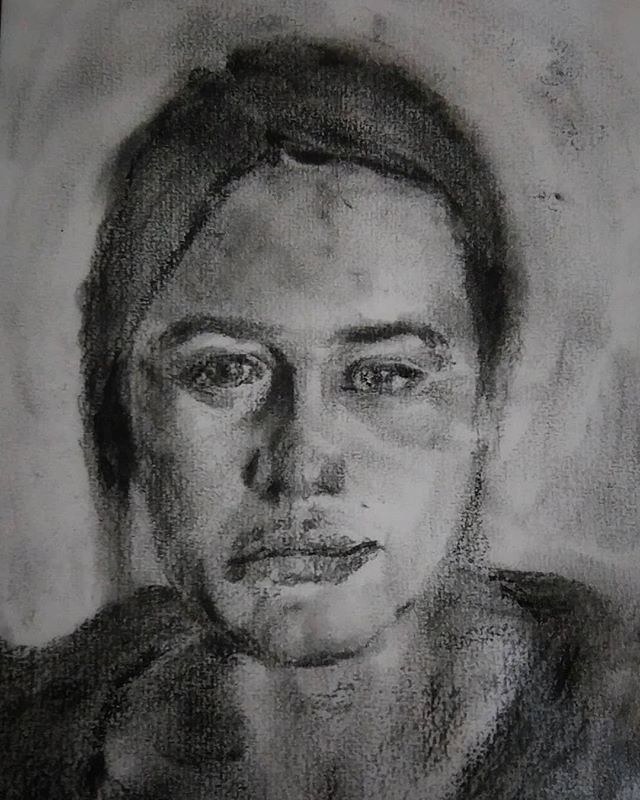The image is a photograph of a detailed pencil and charcoal portrait of a young girl with straight hair, parted on the side and pulled back, revealing her forehead. The portrait is done on parchment-like official drawing paper with a large grain texture. The girl's face, with pronounced shading and blending techniques, depicts an expressive and somewhat asymmetrical appearance. Her lips have shading that makes their shape a bit ambiguous, and her mouth appears slightly uneven, curving up on one side and down on the other. Similarly, her left eye is positioned a bit higher than her right, contributing to the portrait's unique character. The artist has used a significant amount of gray shading on her neck and one side of her face, creating a play of light and shadow that defines her features. Her eyebrows are detailed, complementing her eyes, nose, and oval-shaped face. The portrait extends to show her neck and throat, which blend seamlessly into her shoulders. She is wearing a dark shirt with a wide collar, skillfully rendered in charcoal, adding depth to the dark setting suggested by the surrounding shading.